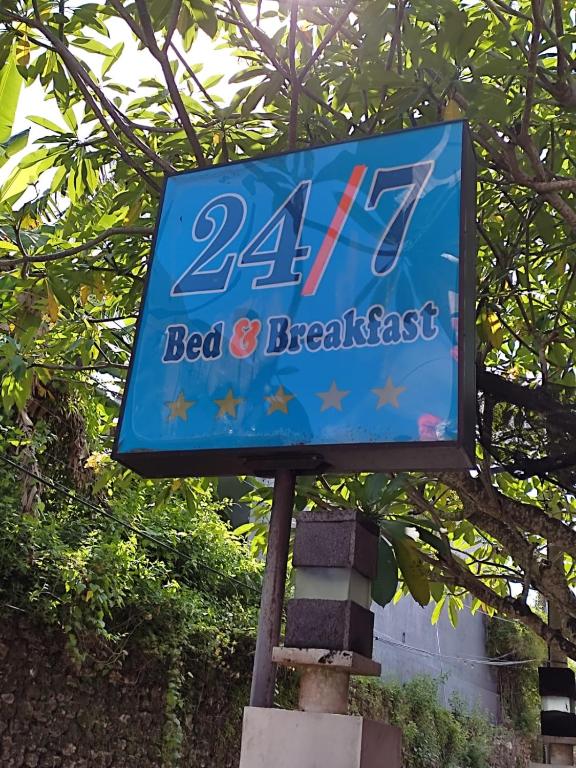The photograph features a prominently displayed bed and breakfast road sign mounted on a sturdy metal pole with a black frame, accompanied by a wooden and concrete post at its base. The sign reads "24/7 Bed & Breakfast" in dark blue and peach-orange lettering against a lighter blue background. Below the text are five gold stars, arranged horizontally. The scene captures a clear, sunny day, with sunlight filtering through the lush, vibrant green trees and bushes in the background, casting dappled shadows on the sign. A closer look reveals a gray stone wall directly behind the sign, partially obscured by a black metal structure and a white stone wall to the right. The low angle of the shot and the proximity to the sign indicate its accessibility.